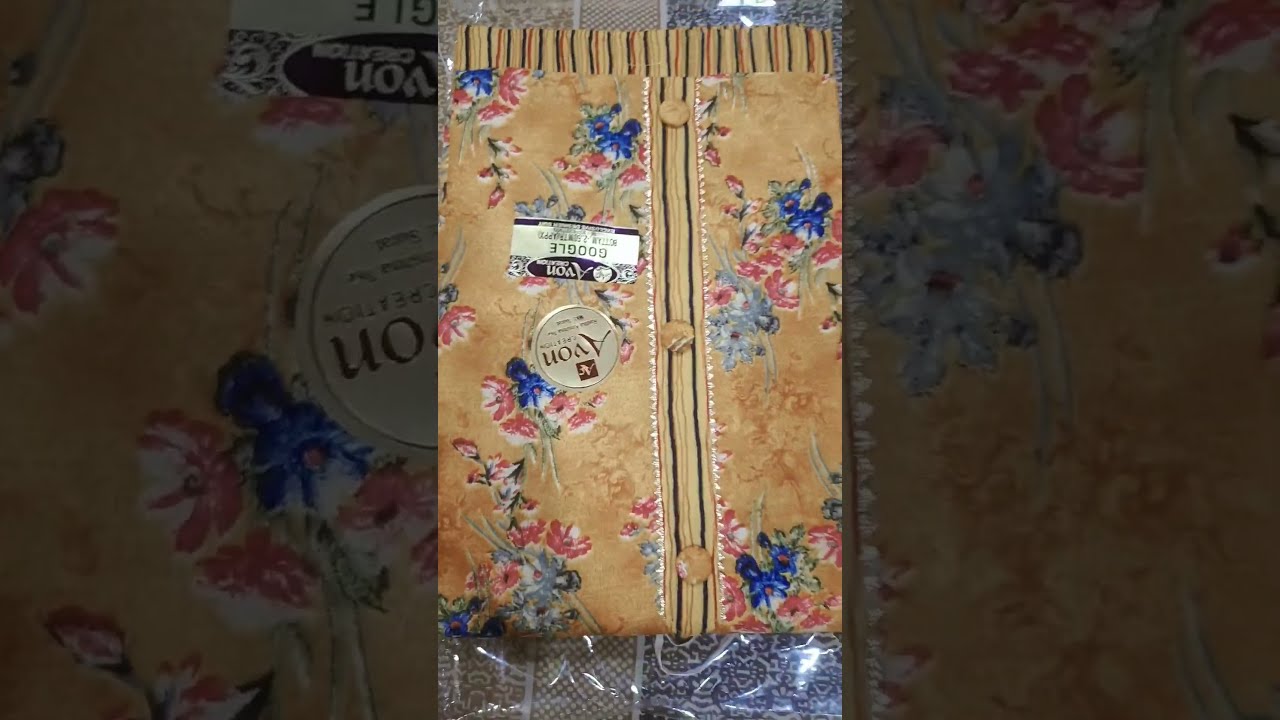The image displays a single object, likely a tan or brown vest or shirt adorned with three buttons, encapsulated in clear plastic packaging. The main visual is centered on a rectangular panel that showcases the fabric's floral pattern, featuring blue and red flowers with green stems. Accompanying this are fragmented, zoomed-in pictures on either side, creating a triptych effect. The object, which takes up most of the frame with only slivers of tablecloth or fabric in the background visible, bears distinctive stickers on its plastic cover. These stickers, gold in color, bear the Avon company name, with one sticker being circular and the other rectangular, positioned upside down on the left side of the item. The photo appears to be a screenshot taken from a mobile device and shared on social media.